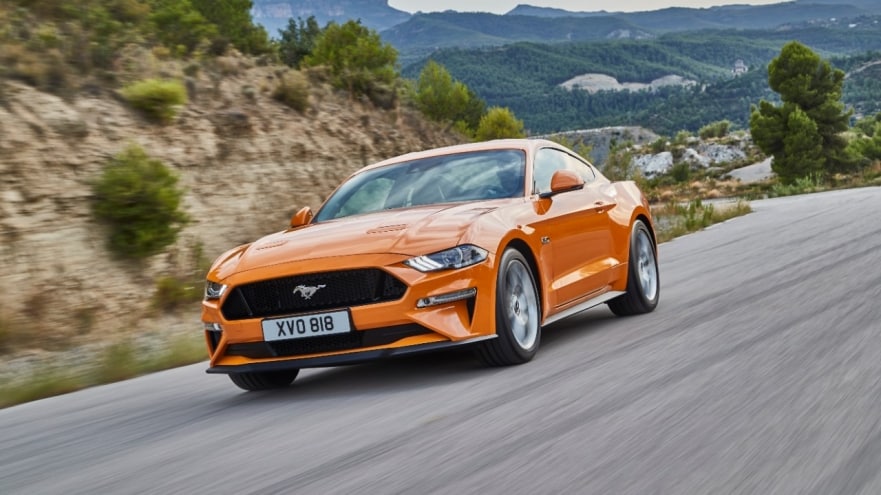The image captures a dynamic scene of a sleek, metallic orange Ford Mustang, emblazoned with its iconic silver running horse logo on the black grille, navigating through winding, mountainous terrain. The car is photographed in motion, suggesting that the shot was taken from another vehicle ahead of it, lending an air of kinetic excitement to the composition. It's a two-door sports car with a European-style, elongated license plate marked "XB-0818," underlining a sense of high-performance elegance. The road, paved and coiling downwards from left to right across the photo, is flanked on one side by a steep brown cliff adorned with green shrubbery and on the other by rolling hills and lush, green forests. The background is a vast expanse of verdant mountains under a clear, daytime sky, indicative of a vibrant spring or summer day. The scene exudes a sense of thrill and freedom, perfectly encapsulating the joy of driving through the captivating, natural landscape.